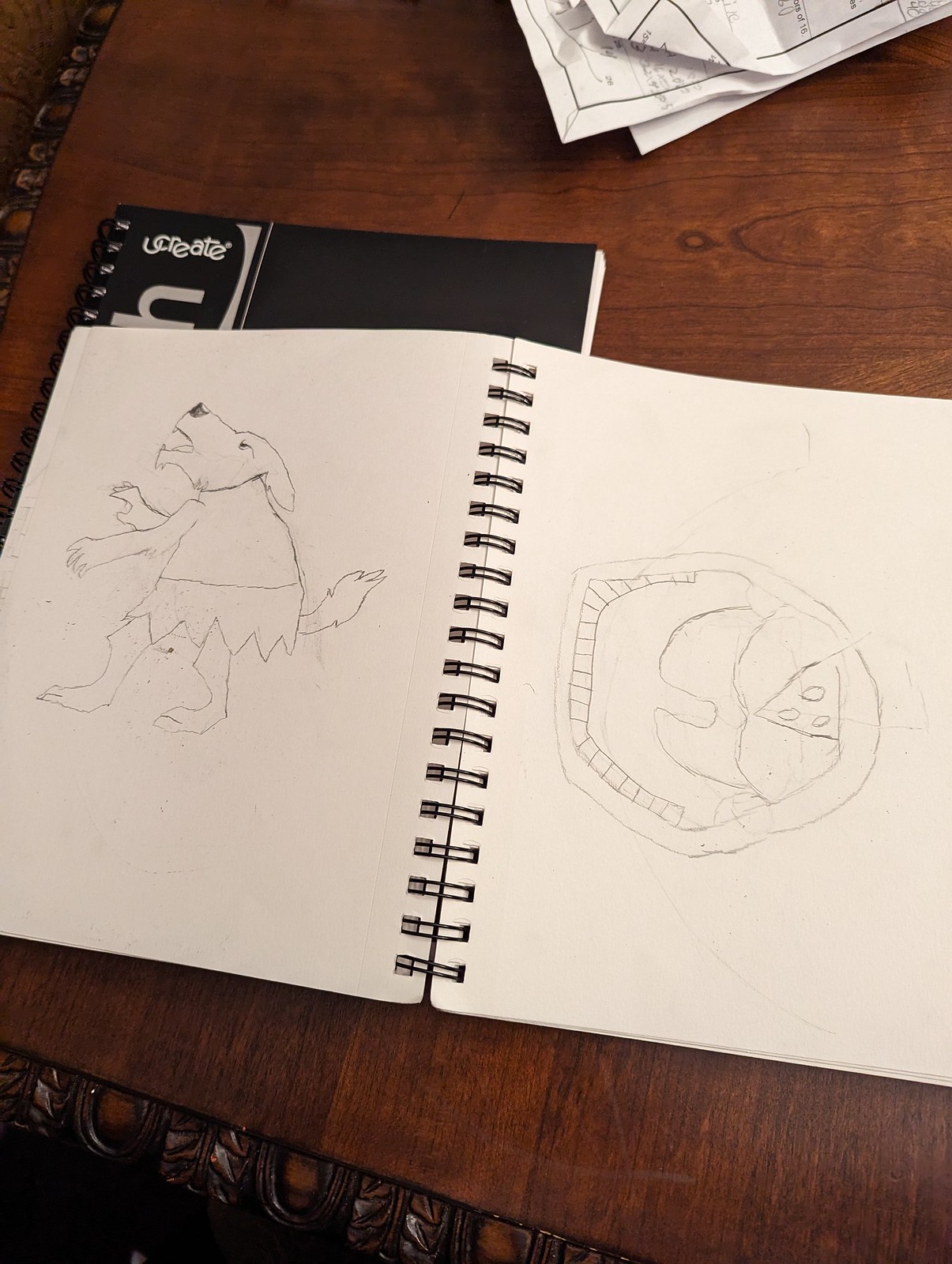In the image, we see a portrait-format photograph looking down on a richly carved, dark wooden table that dominates the background. The table features intricate, ornate trim, particularly noticeable in the lower left and extending toward the center. On the table lies an open spiral notebook with two white pages. The notebook rests atop another closed black spiral notebook, partially visible, with a piece of white text on it that reads “create.” In the upper right corner of the image, there are some loose papers with black text.

On the left page of the open notebook, there's a detailed pencil sketch of an anthropomorphized dog or werewolf standing on its hind legs. The figure is wearing a primitive skirt or loincloth reminiscent of a caveman’s attire and is looking upward with its mouth open, revealing two visible teeth. Its tail extends out from the back of the skirt.

The right page features a more abstract pencil drawing, comprising a couple of disfigured circles incorporating various shapes. The top edge of the main circle is adorned with small square shapes that could be interpreted as teeth, suggesting the drawing may represent an open mouth, complete with a tongue and tonsils.

The combined elements of the detailed carvings of the desk, the layered notebooks, and the intricate doodles create a scene rich in texture and artistic exploration.